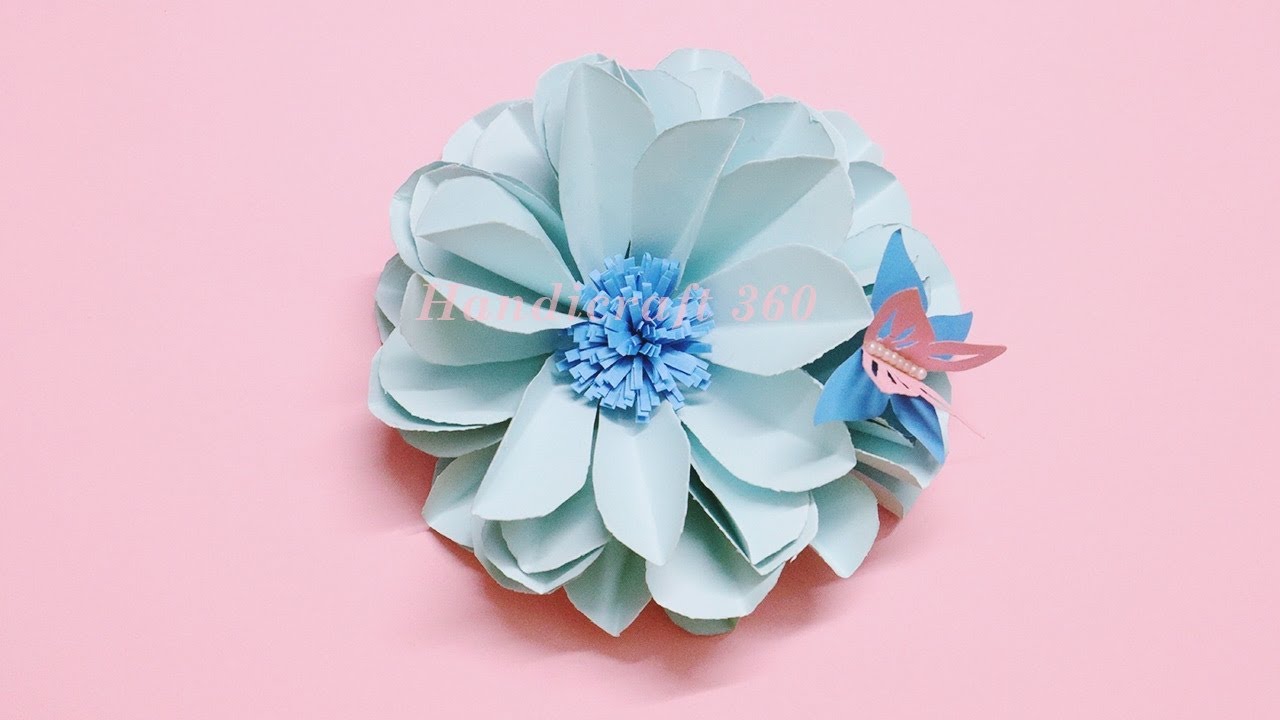The image captures a meticulously crafted paper flower and a delicate paper butterfly, both set against a smooth, solid pastel pink background. The centrally located flower is composed of multiple layers of pastel blue paper petals, resembling the fullness and complexity of a rose. The large outer petals transition into slightly darker blue, narrower strips at the flower's core, adding depth and contrast. To the right of the flower rests a charming butterfly, with blue-outlined lower wings and pink upper wings featuring intricate cut-out shapes that lend additional dimension. The butterfly's body is adorned with a row of pearl-like beads, enhancing its elegance. Imposed over the top of the flower, the text "Handicraft 360" appears slightly transparent, integrating seamlessly with the artwork below. Shadows cast by the flower and butterfly add to the lifelike and three-dimensional appearance of the composition.